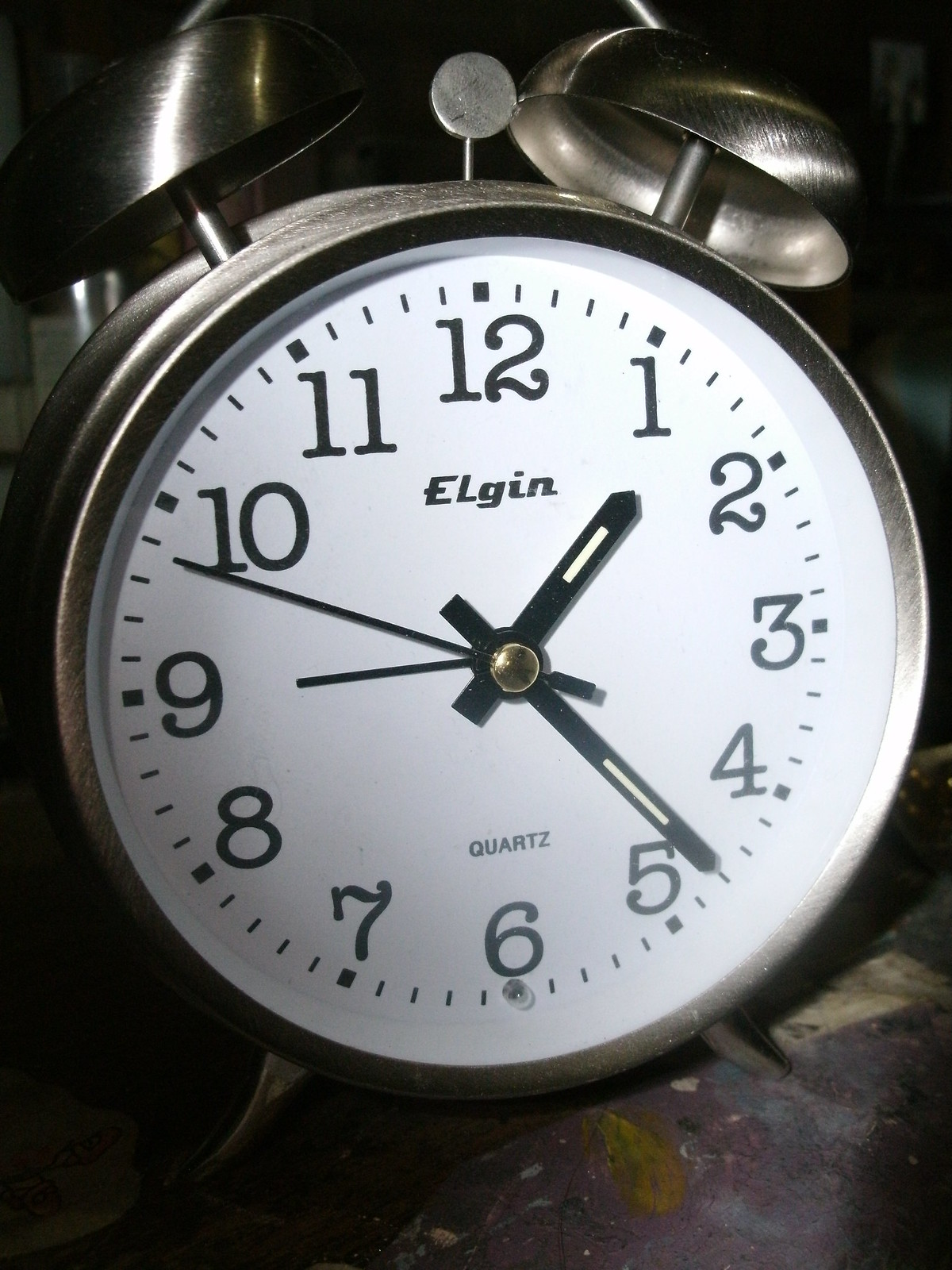This is an up-close, detailed photograph of a vintage Elgin brand alarm clock standing on a grayish surface with hints of blue and yellow paint in the bottom right corner. The clock is slightly tilted to the left, showcasing its metallic silver body and black text on a bright white face. The clock has a classical design with two prominent metal bells on the top, connected by a slim silver piece that facilitates the ringing mechanism. 

Encased within a silver frame, the clock's face features a black border followed by a gray border inside, which encloses the white dial. Black numbers are positioned around the dial, with "Elgin" written just below the number 12 and "Quartz" above the number 6. It displays a precise time of 1:23 and 49 seconds, indicated by short black hour and minute hands, and a thin, elongated second hand. The clock is supported by two small silver feet that give it stability. The striking contrast between the dark background and the bright clock face highlights its detailed structure, making the classical elements and intricate design features prominently stand out.